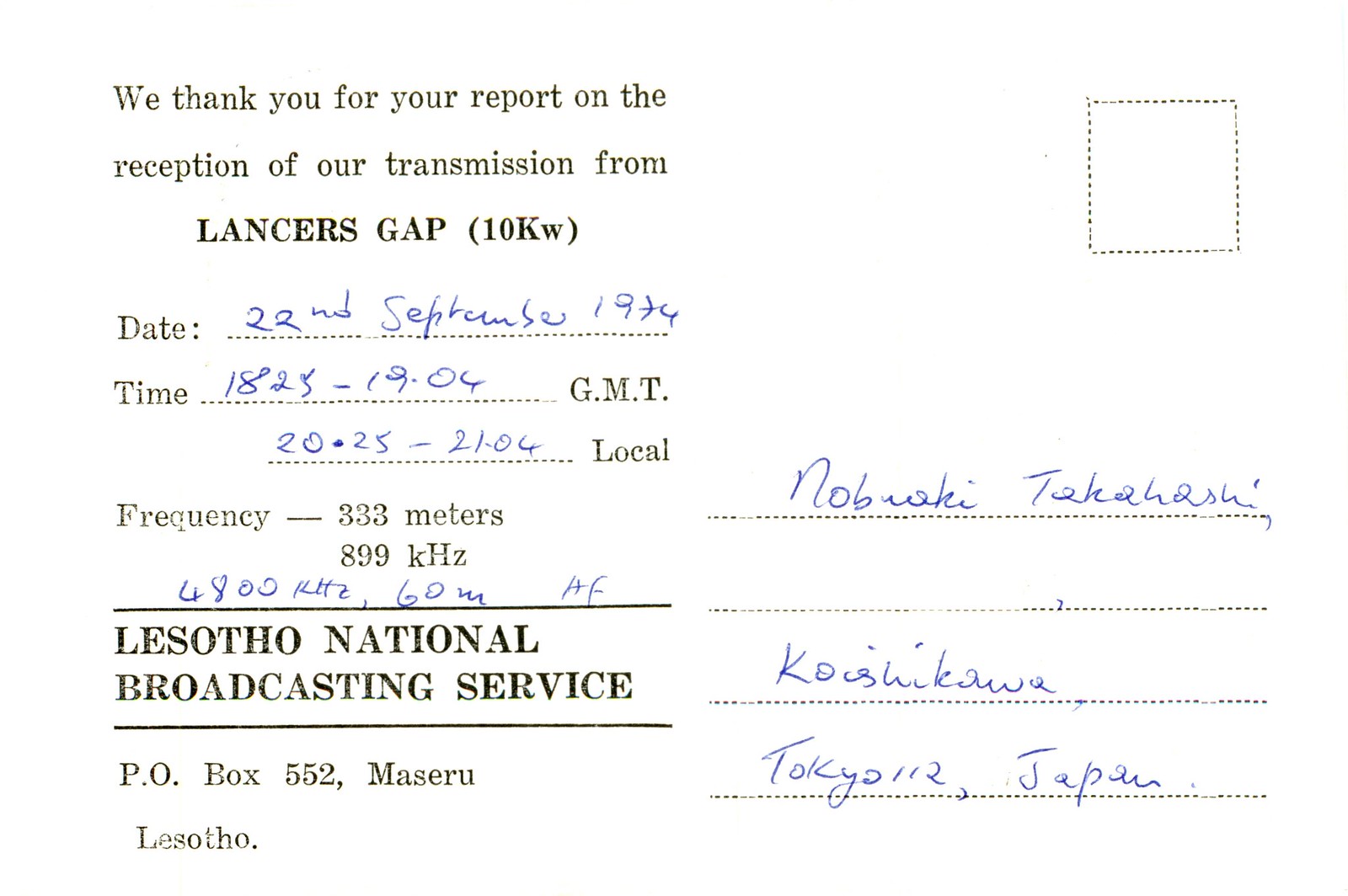The image depicts a form resembling the back of a postcard, utilized as a transmission confirmation document from the Lesotho National Broadcasting Service. At the top in black print, it states: "We thank you for your report on the reception of our transmission from Lancer's Gap (10 kilowatt)." Handwritten details below include "Date: 22nd September 1924, Time: 1825 to 1904 GMT (2025 to 2106 local)," and "Frequency: 33 meters, 899 kilohertz, 6800 kilohertz at 60 meters AF." The form features the address of the Lesotho National Broadcasting Service, P.O. Box 552, Masaru, Lesotho, and contains a return address on the right for Nobuaki Takahashi in Koshihawa, Tokyo, Japan. The document, likely from an era before computers, includes various handwritten details in blue ink, giving it an authentic and vintage appearance. A small dotted square on the top right suggests a placeholder for postage.